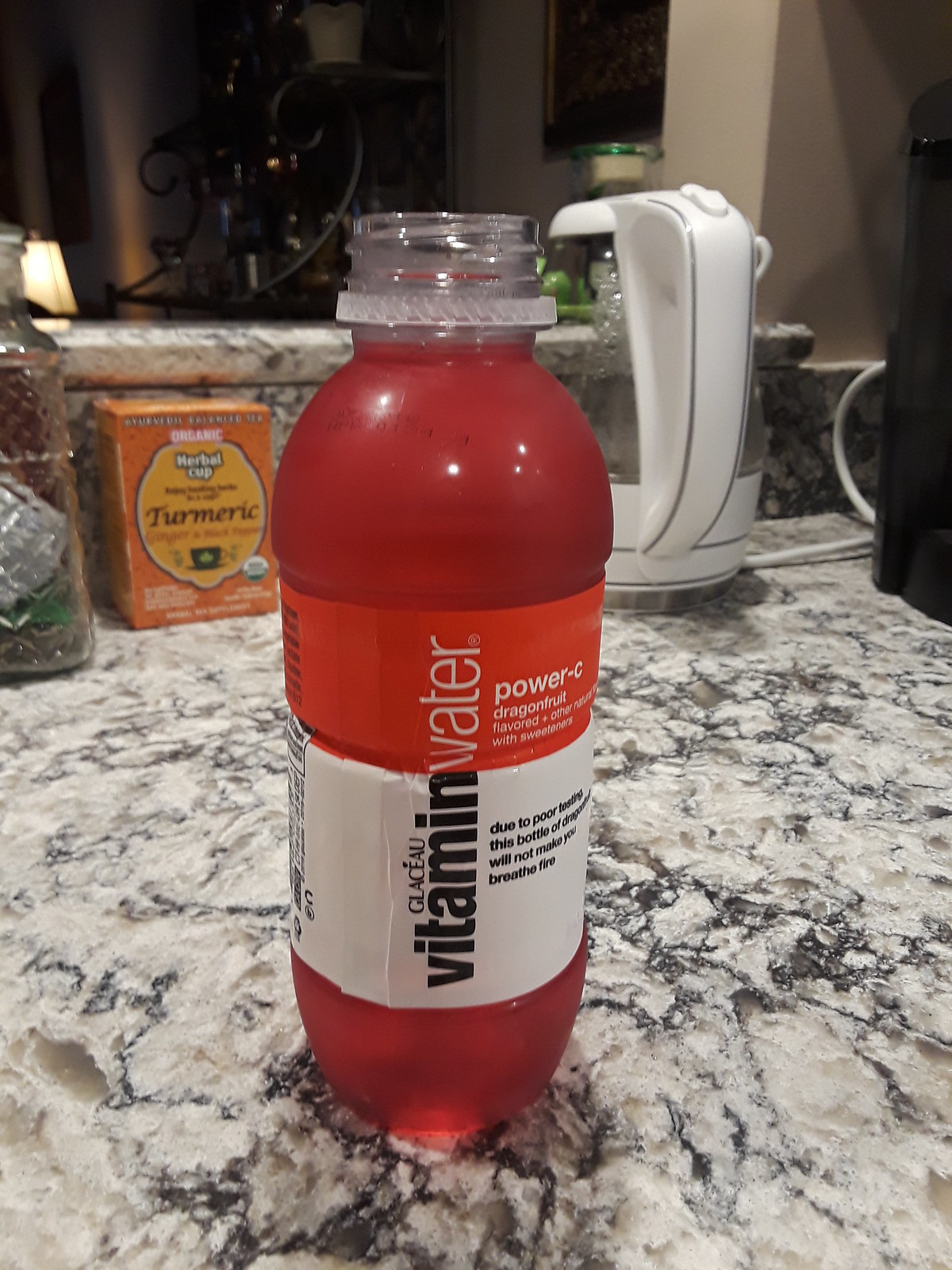The photograph is a vivid, colorful image showcasing a white and gray stone countertop with prominent veining, suggesting it might be granite. On this countertop sits a clear, plastic, open bottle of Vitaminwater filled with a reddish-orange liquid that fades into a lighter tint near the bottom. The bottle is casting a shadow on the countertop. Its label is white at the bottom and transitions to orange at the top, with text indicating something about "Power 2". Additionally, a can opener is visible in the background. To the right, there's a small orange box labeled with turmeric in gold lettering. Beside the turmeric box is a clear glass jar containing tea bags. In the distance, the image captures part of the walls and some wrought iron furniture, adding depth to the scene.